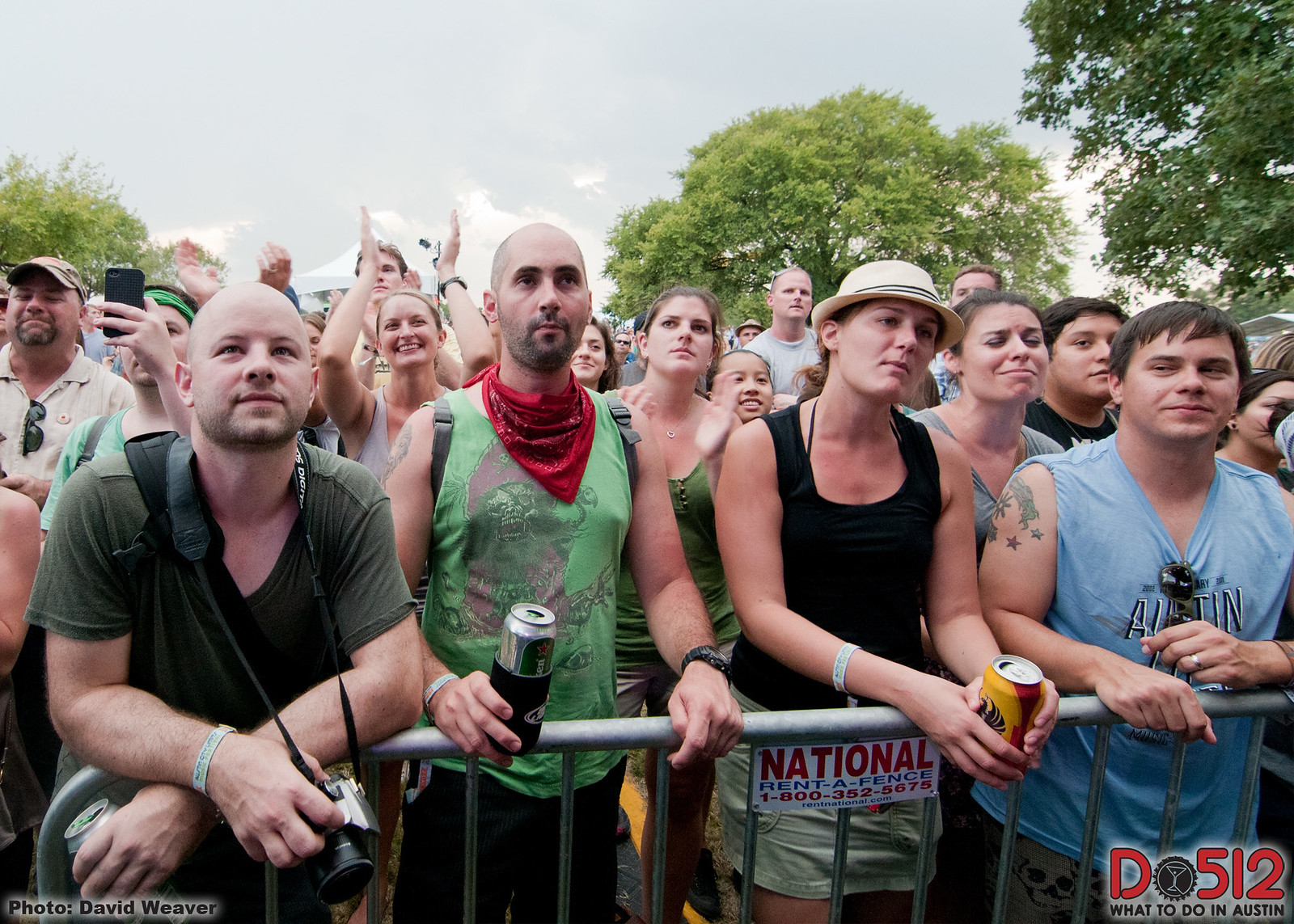This outdoor photograph captures a lively scene of 20 to 30 people standing behind a waist-high metallic fence, marked with a small sign that reads "National Rent-a-Fence 1-800-352-5675." Among this diverse group, composed of both men and women, some individuals are smiling and appear to be enjoying a festive atmosphere that suggests they might be at a concert. Trees in the background enhance the natural setting, while the blue sky dotted with clouds adds to the overall cheerful mood. The front row is particularly detailed: one man with a green short-sleeved shirt, a bracelet, and a camera; another man holding a drink and wearing a red bandana; a woman with a hat and a drink; and another man with sunglasses tucked into his shirt. Hands rest casually on the fence, indicating a relaxed vibe. Notably, the bottom left corner of the image credits the photo to David Weaver, while the bottom right corner features "DO512 What to do in Austin" accompanied by a logo with a drink in a black circle.